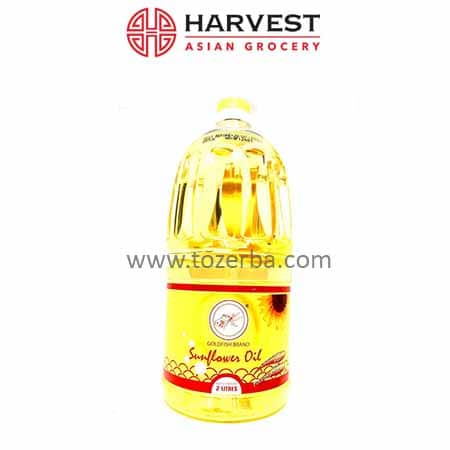The image showcases a two-liter clear plastic bottle of Sunflower Oil against a stark white background, making the product appear to float. The bottle contains a golden yellow liquid and features a yellow cap. The prominent yellow label on the front displays 'Sunflower Oil' in cursive red text. Above this, there's a logo, possibly picturing a sunflower, and at the very top of the label, the brand 'Harvest Asian Grocery' is written, accompanied by an oriental-style red circular emblem split into two halves. Additionally, a small white circle on the label contains a koi fish emblem. Overlaying the middle of the image is the watermark 'www.tozerba.com' in light gray.